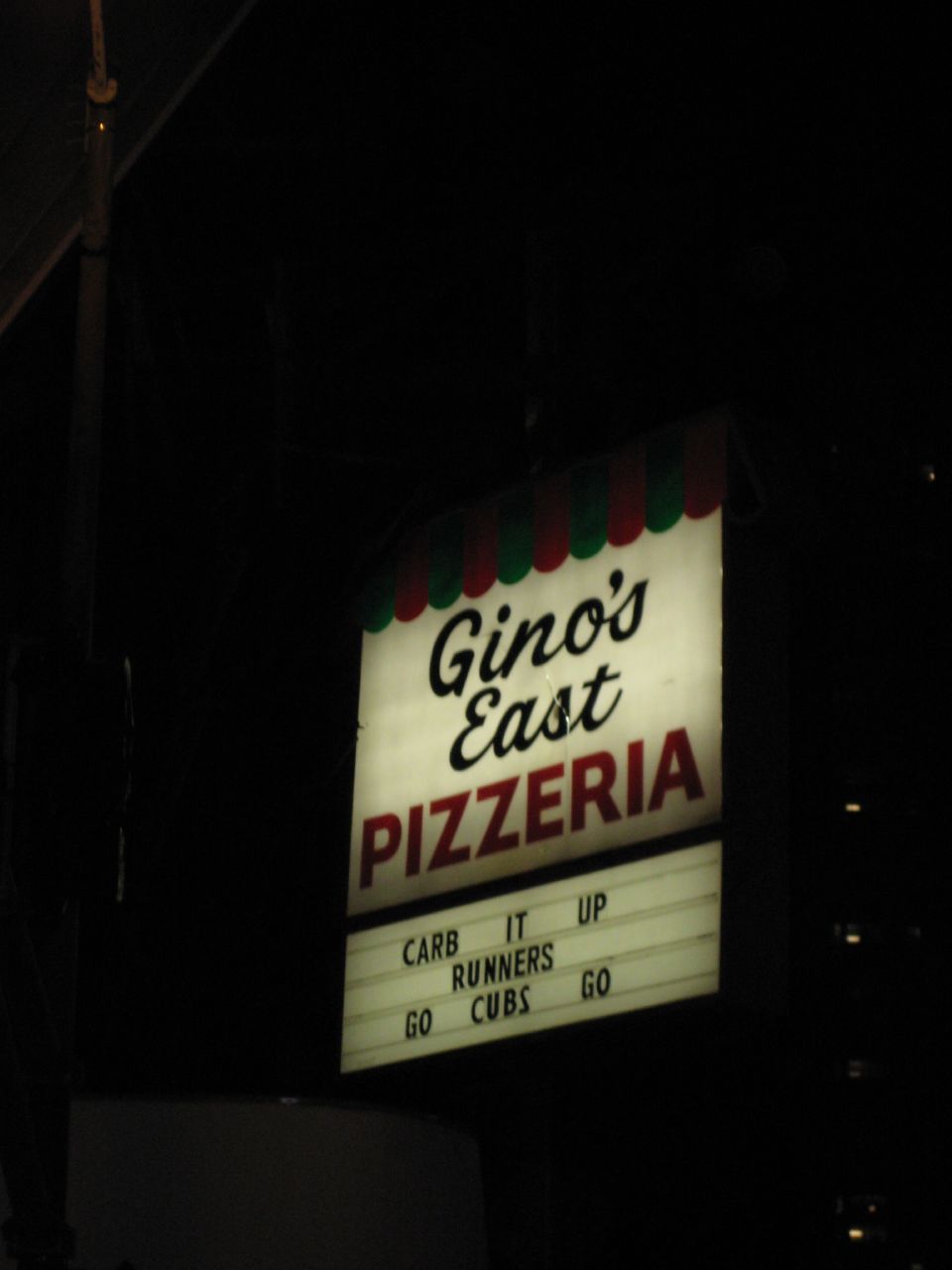In this nighttime photograph, the focal point is a brightly illuminated sign for Geno's East Pizzeria, positioned centrally against a nearly pitch-black background. The sign itself has a white background with "Geno's East" prominently displayed in elegant black cursive, while "PIZZERIA" is written in bold red capital letters below it. Adding a festive touch, the top of the sign features scalloped borders with alternating red and green stripes. Beneath the main sign, a smaller rectangular section contains changeable text, currently reading, "CARB IT UP", "RUNNERS", and "GO CUBS GO", each on separate lines in black text. A pole is slightly visible in the top left corner, and some house lights can faintly be seen in the background, contributing to the nighttime ambiance of the scene.